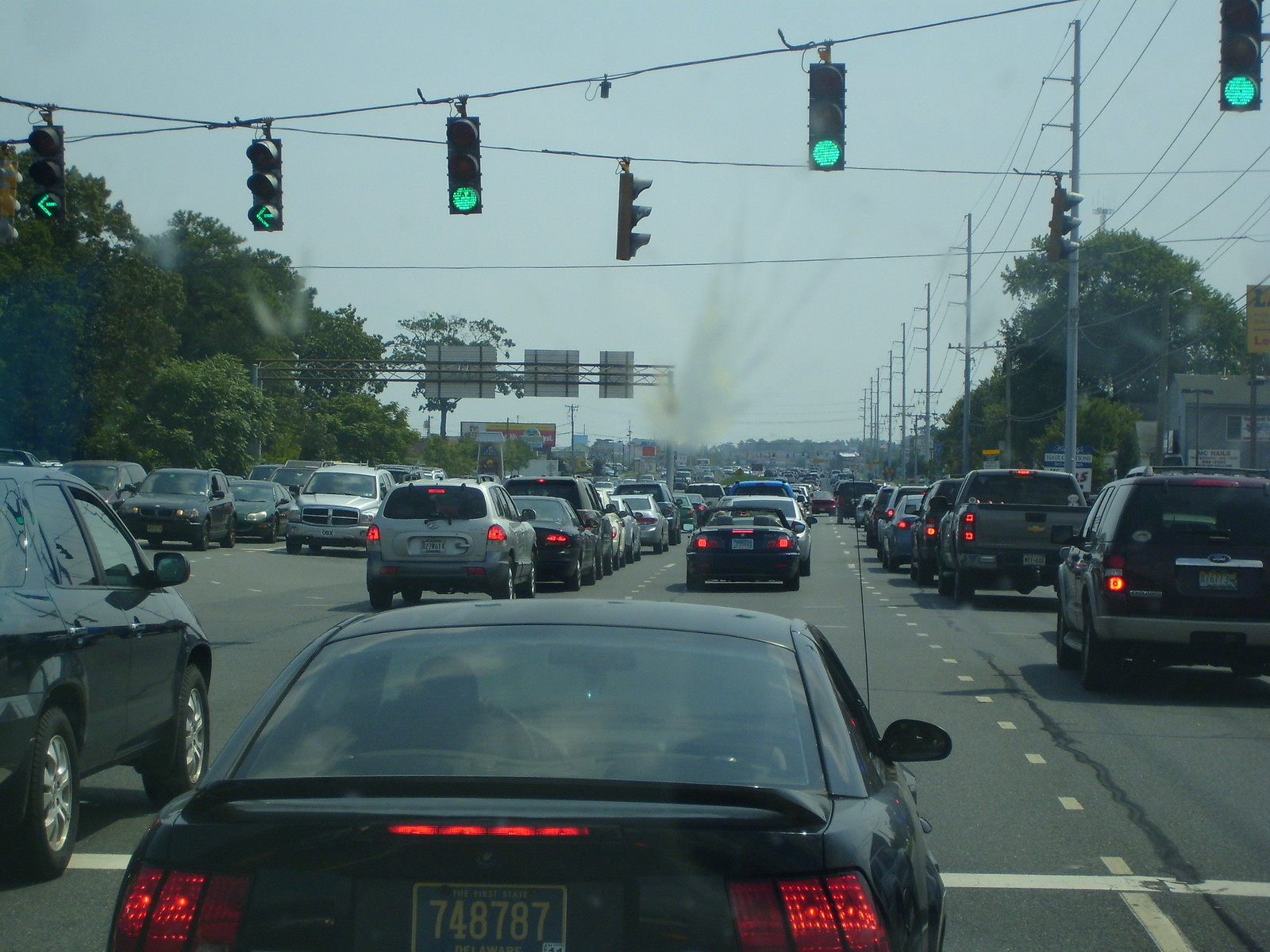The slightly rectangular horizontal image captures a congested urban scene through a vehicle windshield. A line of green traffic lights spans the top diagonally from the lower left to the upper right, indicating the go signal despite the heavy traffic. Below these lights, the roadway is crowded with vehicles in all three lanes moving in the same direction as the photographer. The red glow of brake lights pervades the scene, highlighting the bumper-to-bumper traffic. On the left side of the frame, three additional lanes teem with vehicles heading in the opposite direction, revealing the front view of their cars. Dominating the center of the background, a column of smoke rises, casting a sense of unease over the bustling traffic.